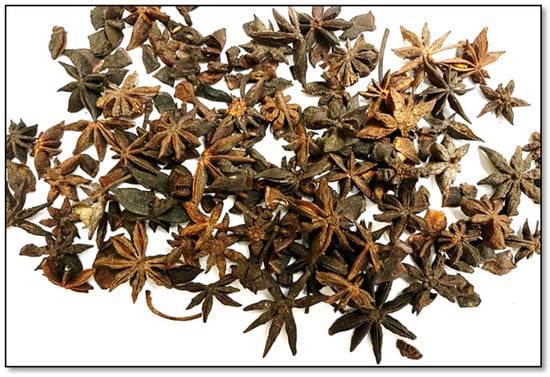This image presents a captivating collection of preserved star-shaped leaves, meticulously arranged against a stark white background. The leaves exhibit a range of colors from greenish tones to shades of brown, with some appearing almost black or gold. Each leaf roughly measures five to eight points, with varying sizes that evoke a resemblance to starfish. Several leaves display an intriguing texture that mimics stone or metal. Scattered randomly across the middle three-quarters of the image, the leaves create a visually engaging pattern, leaving the corners blank and emphasizing the central assortment. The drying and preservation of these leaves underline their delicate beauty, enhanced by occasional orange flowers and stems interspersed among them. The collection, comprising around a hundred leaves, highlights the meticulous care and time dedicated to this enchanting botanical display.